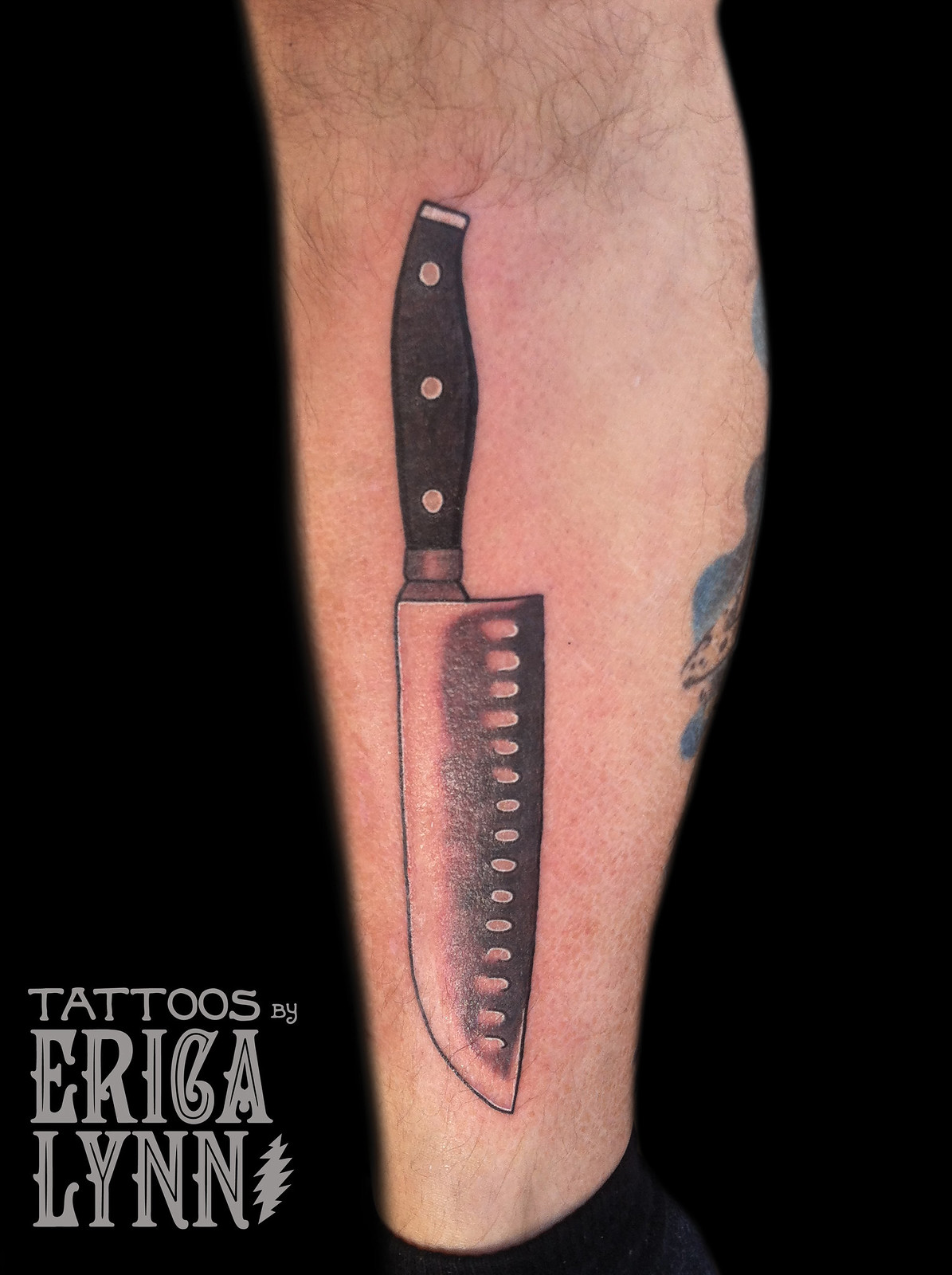The image is a detailed color photograph of the side of a male's leg, specifically showcasing his calf against a black background. The leg, featuring white skin that has been recently shaved, displays a fresh, photorealistic black and white tattoo of a chef's knife. The knife is positioned vertically along the side of the calf, with the blade running downward towards the ankle. The handle of the knife is black, curved, and features three metal screws, reflecting a wood texture. The blade is wide at the top and tapers toward the bottom, mimicking the appearance of a butcher's knife. Along the sharp edge of the blade are a row of holes, adding to the knife’s realistic depiction. The tattoo has shading that makes the blade appear semi-reflective, enhancing its photorealistic quality. Additionally, there is another bluish tattoo partially visible on the backside of the calf. In the bottom left corner of the image, a white graphic reads "Tattoos by Erica Lynn." This text is in large, all-caps, outlined lettering, with a lightning symbol beside "Lynn." The overall style of the knife tattoo is photographic representationalism realism.